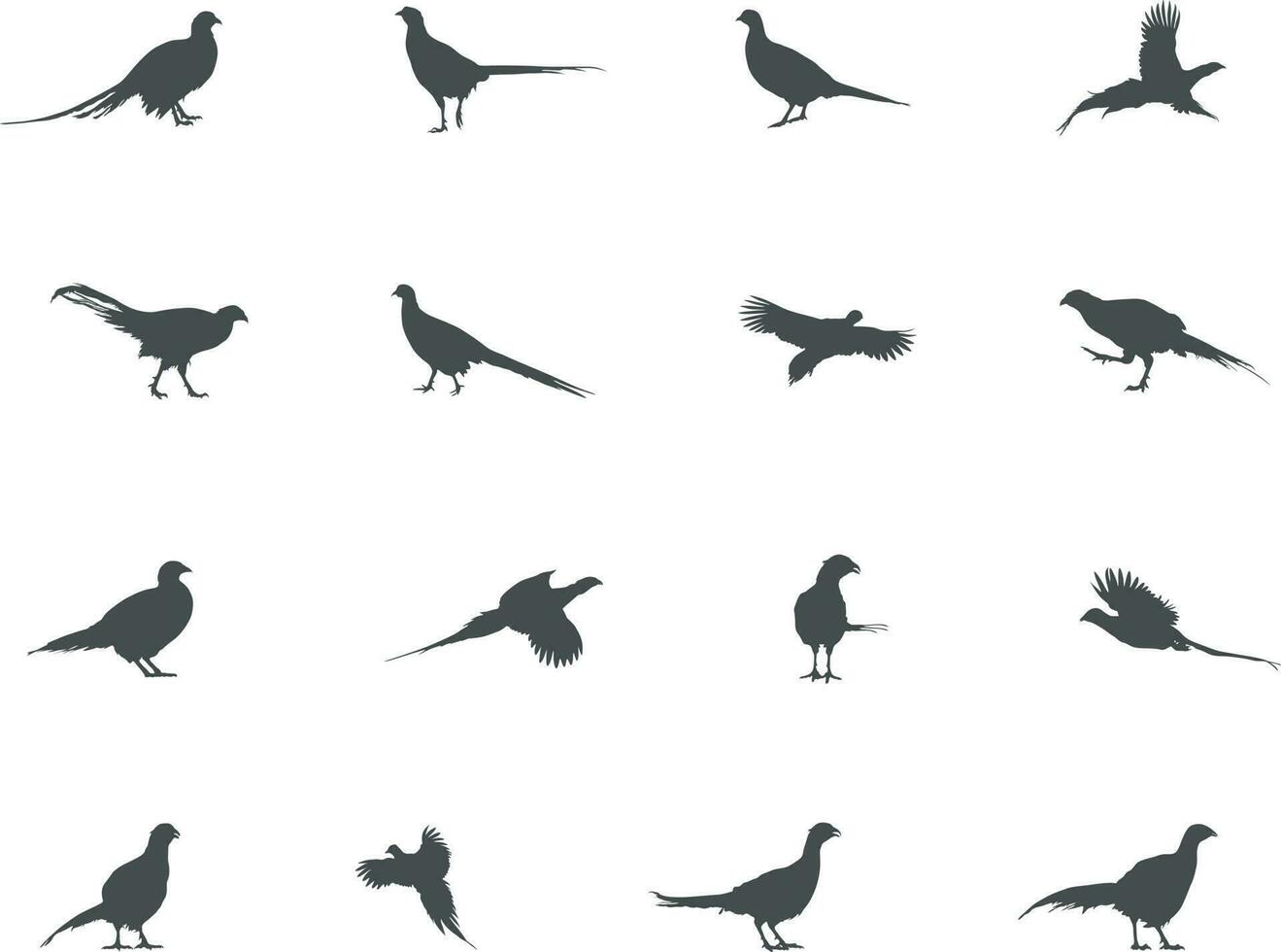The image depicts a series of 16 graphic illustrations of birds set against a stark white background, organized into four rows and four columns. Each bird is presented in varying postures – flying, landing, or standing – and is uniformly rendered in shades of gray. Notable features among these birds include long tail feathers and extended necks, with some exhibiting distinct characteristics such as a small feather tuft rising from the head. The birds’ positions are diverse: some face each other, some appear in flight with their wings extended, and others stand with one foot raised. The uppermost bird in the first column is a turkey, while other birds resemble peacocks, hawks, and crows, showing a variety distinct poses and tail orientations. Though the specific species are ambiguous due to the grayscale rendition, the birds share structural similarities, particularly in tail and neck morphology, hinting at possible pigeon family characteristics.